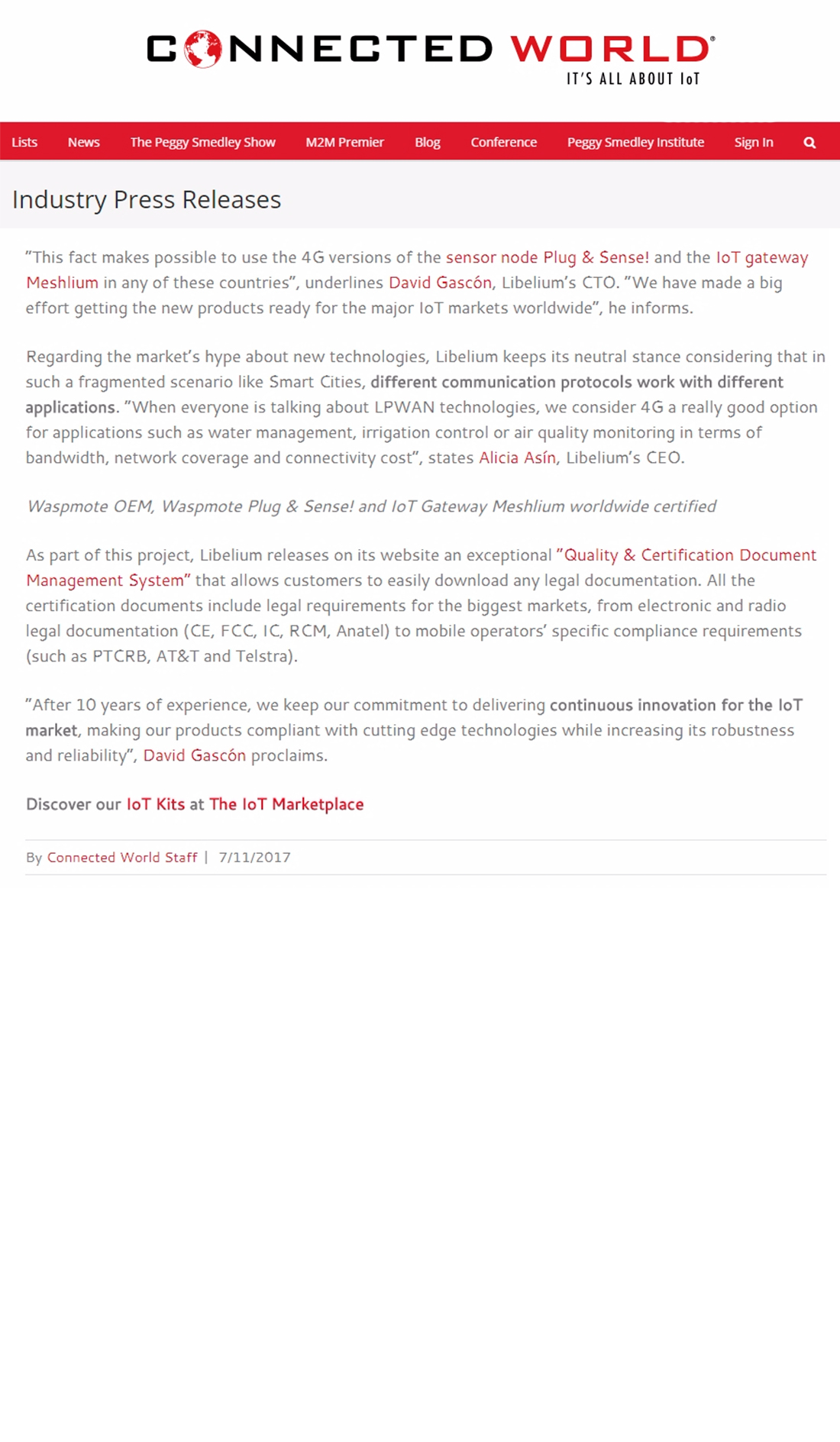The website by Connected World features a prominent red header with navigational options, though most are in less legible white text, with the exceptions of "Sign In" and "News" on the right side. The title "Connected World" includes a stylized 'O' represented by a red image of the globe, where "Connected" is in black and "World" is in red. Below this header, a gray bar indicates "Industry Press Releases". The main content discusses the usability of 4G versions of various sensor nodes, plugs, and sense devices, emphasizing neutrality regarding technology and communication protocols within smart cities, expressing that such fragmentation doesn't hinder their applications. The text continues to state the company's decade-long commitment to innovation and product compliance with advanced technologies. A highlighted quote by David Casson in red invites readers to "Discover our IoT kits at the IoT Marketplace." Finally, the article is credited to the Connected World staff with a publication date of July 11, 2017.